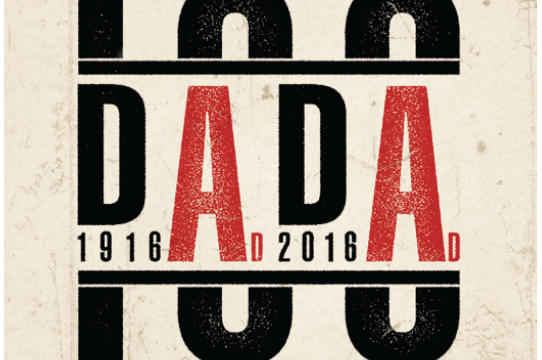This rectangular poster, wider than it is tall, has a cream-colored background with light gray mottling. Central to the design are large alphanumeric characters and decorative elements in black and red. In the middle of the poster, it prominently displays "D.A.D.A." Each "A" is an oversized red capital letter, significantly larger than the black capital "D" letters positioned next to them.

Below the first "D," with the base aligned but slightly indented to the right, is the date "1916" in black. The second "D" has the date "2016" below it, similarly positioned, with each digit, except the trailing "6," directly beneath the "D.” The dates and "D" characters are consistently black, whereas the "A" characters are bright red and occupy considerably more vertical space.

A thick black line runs horizontally above and below the "D.A.D.A" text. Suspended above this line, a bold black vertical column caps the first "D." An upside-down thick "U" shape connects above the letters "A" and the final "D". Similarly, directly beneath the lower black line, each "A" is supported by a thick right-side-up "U," aligning perfectly with the inverted "U" above.

The overall font style is noted for its length over width, giving the text a slender appearance. The tactile design and color contrast—cream background, black and red letters—make the poster strikingly visual and rhetorically powerful, capturing the eye with its asymmetric letter sizing and harmonious geometric patterns.